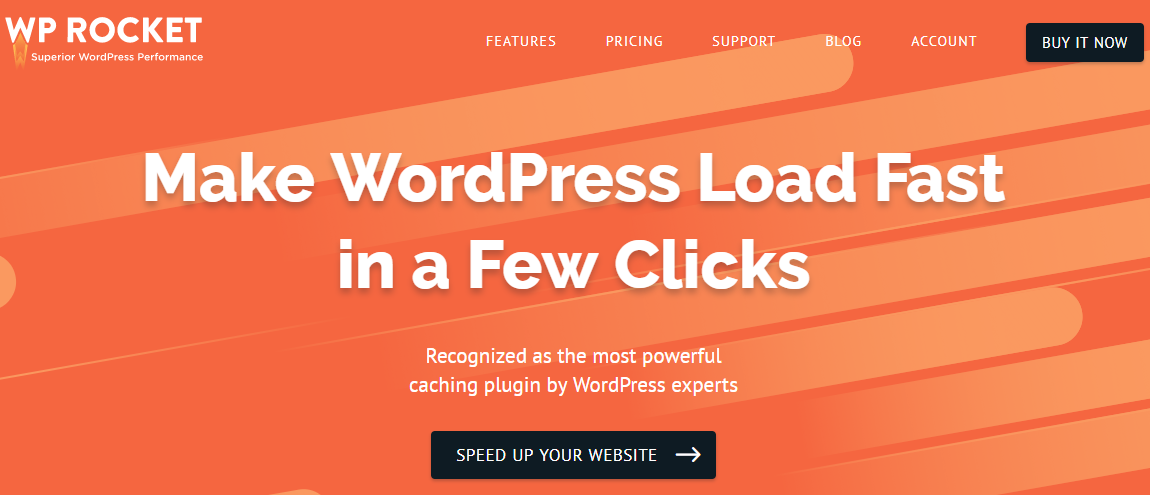The rectangular image, oriented with its longer side running horizontally, features a predominantly orange background with varying shades. In the upper left corner, bold text reads "WP Rocket," and just below, it states "Superior WordPress Performance." 

In the upper central part of the image, starting from approximately the middle, the navigation options are listed: "Features," "Pricing," "Support," "Blog," and "Account." On the far right, a black box with white text commands attention with the inscription "Buy It Now." 

Centrally placed within the image, large text announces, "Make WordPress Load Fast in a Few Clicks." Beneath this, smaller text proclaims, "Recognized as the Most Powerful Caching Plugin by WordPress Experts." 

Lower in the image, another black box with white text invites action with, "Speed Up Your Website," paired with a rightward arrow.

The design also incorporates stylistic elements: streaks of lighter orange lines diagonally traverse the image from the lower left to the upper right, adding dynamic movement and visual interest.